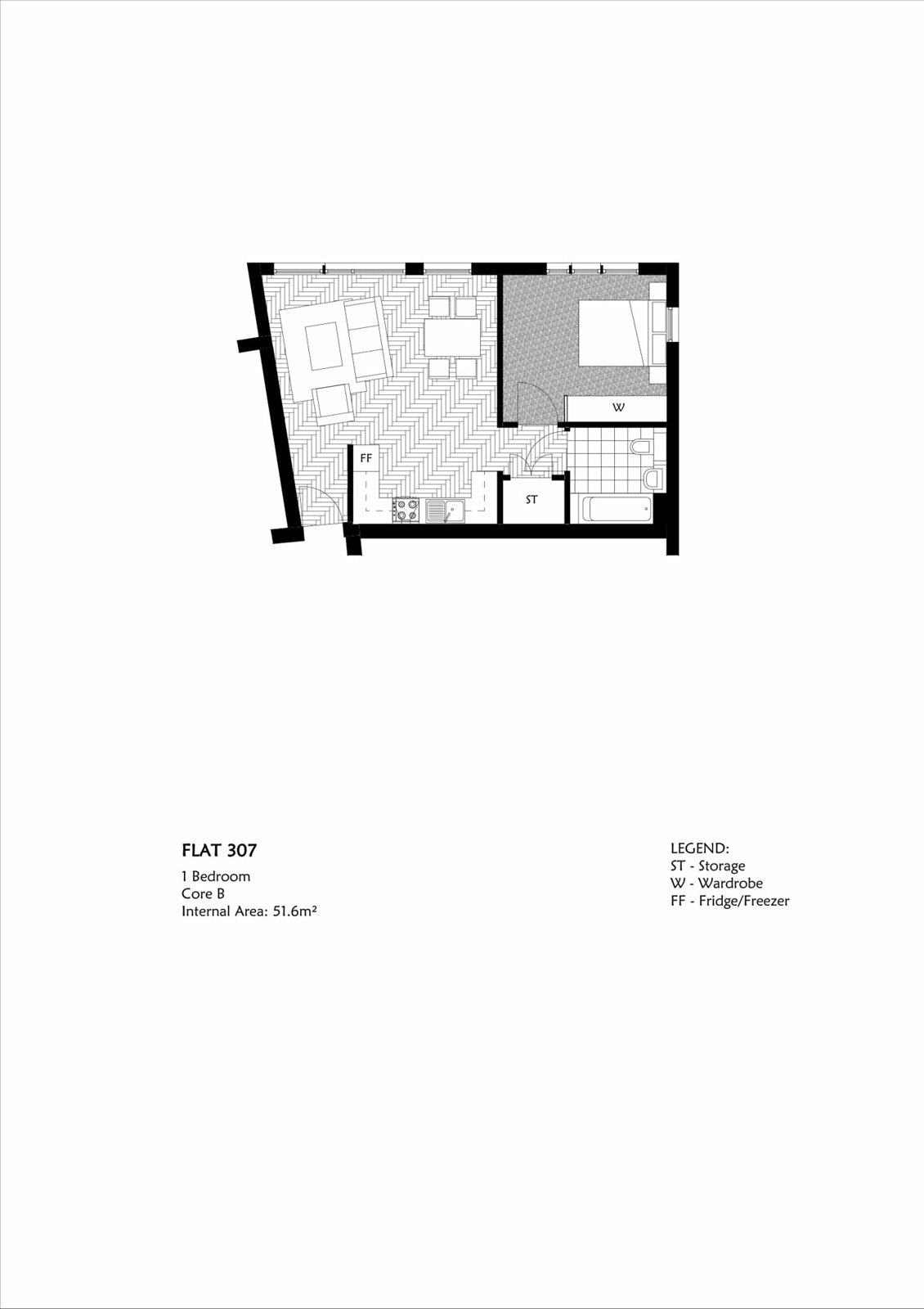This black-and-white blueprint depicts the layout of an apartment, specifically "Flat 307." The design follows a square format with dark black edges and occasional white patches. The text beneath the image reads: "Flat 307, one bedroom, Core B, internal area 51.6 m²." Another section of the text explains a legend for the abbreviations used: "ST" for storage, "W" for wardrobe, and "FF" for fridge or freezer.

At the top of the blueprint, you can see how all the rooms are divided and clearly labeled. On the right side, the label "W" indicates the location of the wardrobe. At the bottom of the blueprint, "ST" marks the storage area. The label "FF" points to the corner where the fridge or freezer is situated. The meticulous detail in labeling and partitioning provides a comprehensive understanding of the apartment's internal structure.